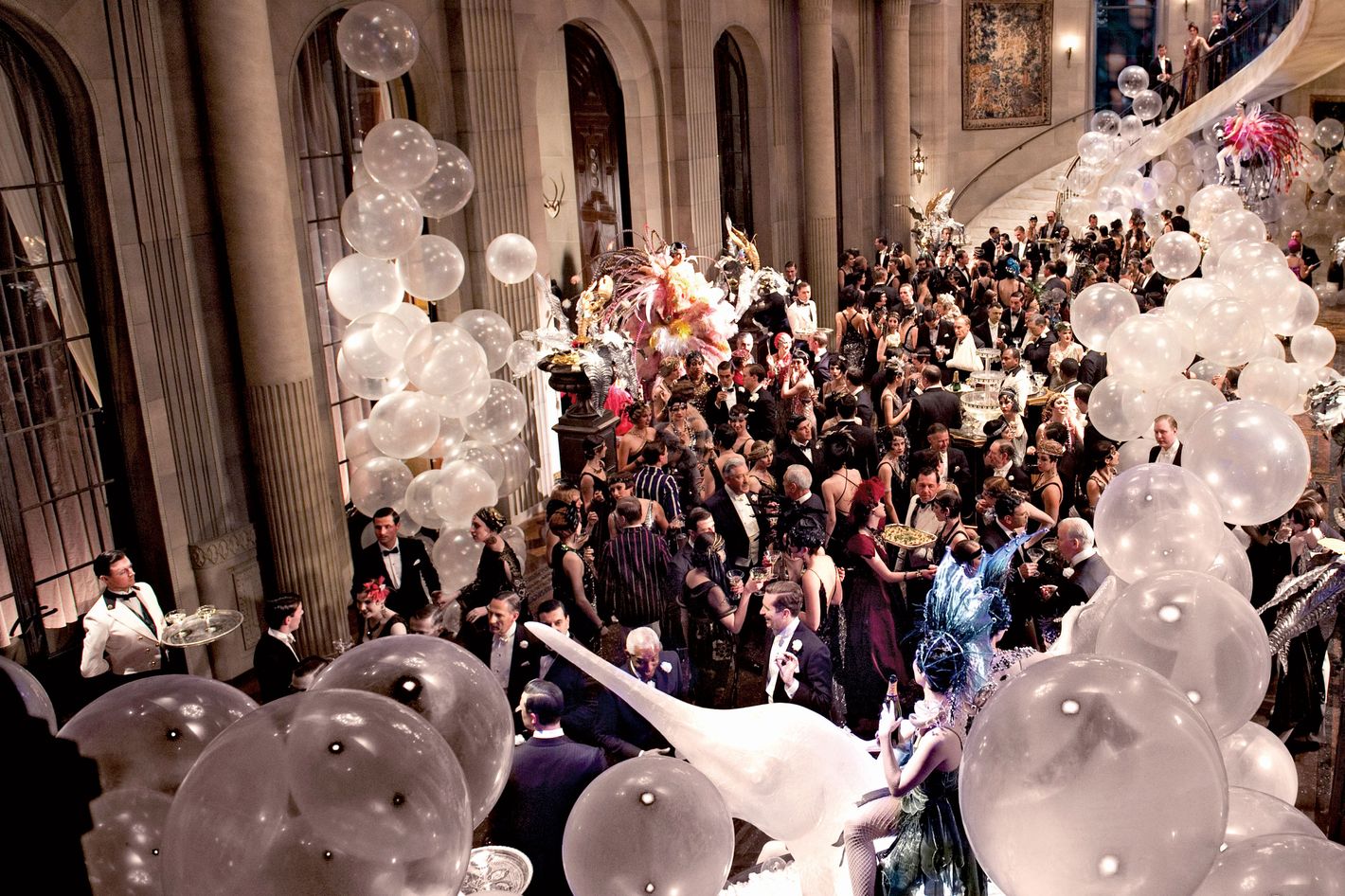The photograph captures a lively and extravagant celebration set in a grand venue with an expansive event hall, likely an estate or lavish theater with high ceilings and columns. The aerial shot reveals a densely packed crowd of hundreds of guests mingling in a large space adorned with white balloons and other festive party favors. A prominent marble staircase winds down on one side, while a large French or European tapestry decorates the wall.

Attendees are elegantly dressed in tuxedos, suits, gowns, and costumes, creating an opulent atmosphere. Many women are dressed as flappers, complete with feathered headdresses, reminiscent of the 1920s or 1930s, while men sport striped jackets and black coats with tails, suggesting a possible 1920s theme or costume party. Among the guests, a woman can be seen riding a white elephant statue, likely part of the event's entertainment.

The scene is further enriched by several butlers and waiters in white coats and black vests, circulating with trays of food and drinks, ensuring the guests are well attended to. The overall ambiance is one of joy and elegance, indicating a special occasion such as a New Year's Eve party or another significant celebration where everyone is enjoying themselves, chit-chatting, and reveling in the festive mood.